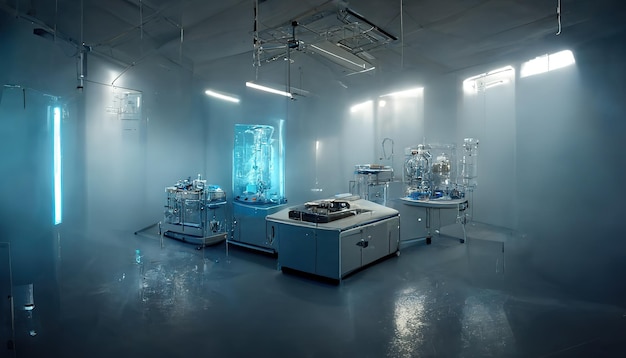The image depicts an eerie, high-tech laboratory room with an industrial design, featuring mist or smoke permeating the air. The room is defined by its white walls and high ceiling, with windows positioned at the very top allowing light to filter in. Fluorescent and suspended halogen lights illuminate the space, adding to its clinical ambiance. On the left side, there are long white cabinets alongside a smaller cabinet containing a blue cylinder filled with intricate machinery. Centered in the room are white tables with white drawers, housing equipment, some of which have glass window displays. There are also carts load with glass apparatuses and wires, suggesting complex mechanical setups potentially for medical use. The shiny, gray floor, appearing almost wet, reflects the lights above, likely due to water misting down from the ceiling. This meticulously detailed and high-resolution photograph creates an atmosphere reminiscent of a scene from a high-tech medical facility or a futuristic video game stage.